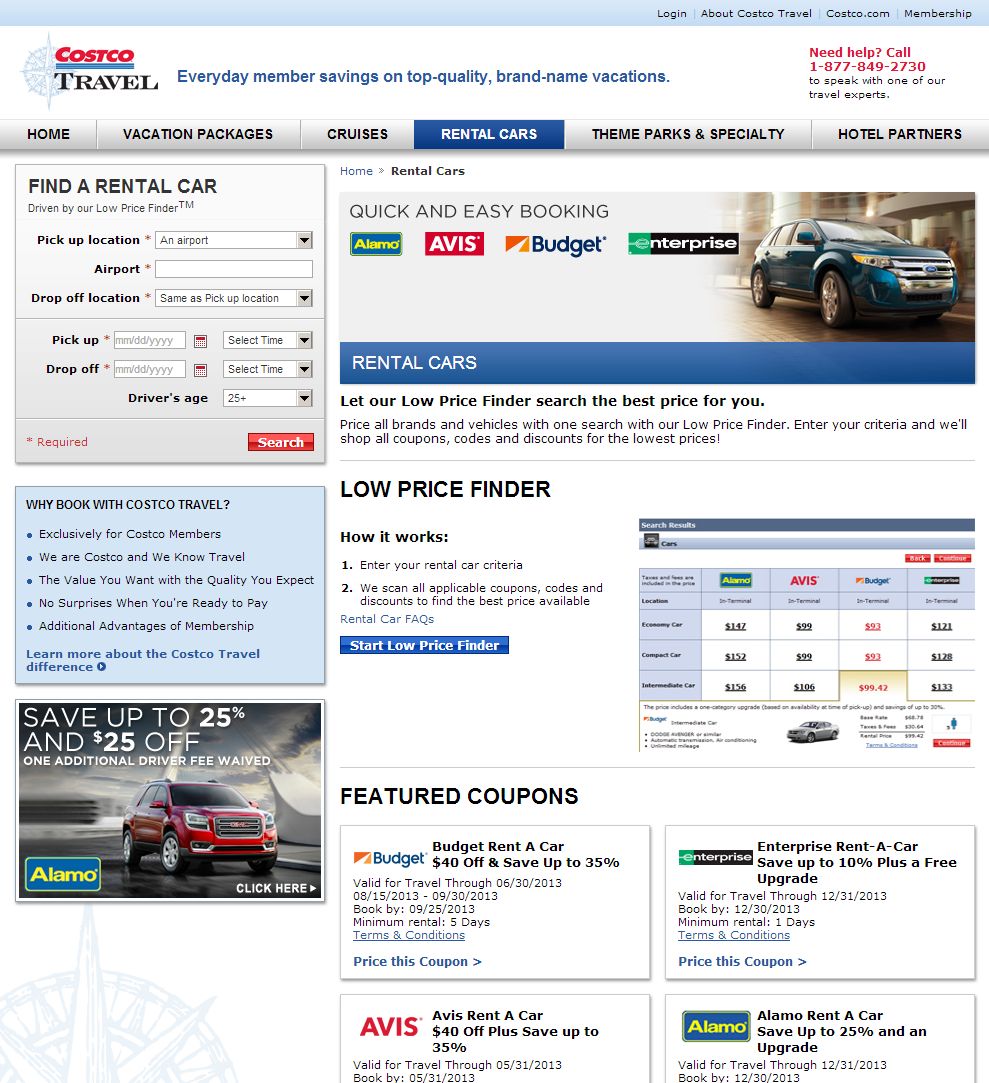This screenshot of the Costco Travel website showcases the exclusive savings and high-quality vacation options available to members. It prominently displays a contact number, 1-877-849-2730, for assistance. The website offers various travel services, including vacation packages, cruises, rental cars, theme parks, and special hotel partnerships. 

On the left side, there's a section labeled "Find a Rental Car: Driven by Our Low-Price Finder," where users can input their pick-up and drop-off locations and times, although these fields are currently blank. The default options include a pick-up from an airport, indicating a focus on convenience for travelers.

Highlighted in blue is the rental car section, with a special note boasting that Costco Travel members can save up to 25% and have the additional driver fee waived with Alamo. A red GMC Terrain and a Ford Explorer are featured to indicate the types of vehicles available.

For rental car booking, the website supports Alamo, Avis, Budget, and Enterprise, each offering different price points for economy and compact cars. An economy car rental with Alamo starts at $47, while Enterprise's lowest is $121. Compact cars have varied rates, with Budget's rate marked at $99.42, noted as a particularly affordable option. 

Additionally, there's an assortment of coupons for further savings. Budget Rent-A-Car offers $40 off and up to 35% savings for rentals of five days or more, with similar promotions available from Enterprise, Avis, and Alamo.

This image underscores Costco Travel's commitment to offering its members valuable, high-quality travel experiences with substantial savings.